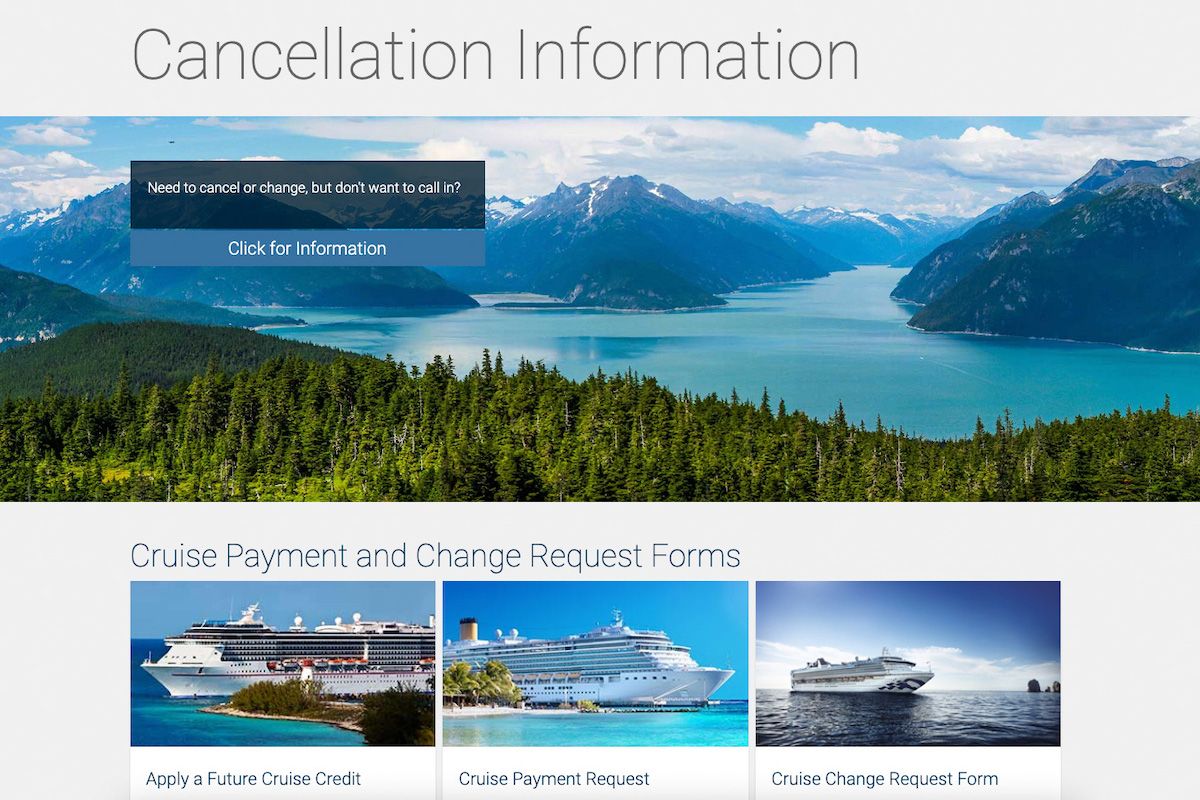A serene landscape shows majestic mountains mirrored in a pristine blue lake under a sky dotted with white fluffy clouds. Lush green trees and grass line the water's edge, enhancing the tranquil scene. Below this picturesque image, there are forms titled "Cruise Payment" and "Change Request." Adjacent to this natural splendor, a large white cruise ship sails across a vast, deep blue ocean. The caption mentions opportunities to apply a future cruise credit and submit cruise payment requests as well as change request forms. The background continues with images of islands adorned with numerous trees and sandy beaches. Multiple mentions of the "Big white cruise ship in a blue ocean" reiterate the availability of cruise change request forms, emphasizing the seamless process for prospective travelers.